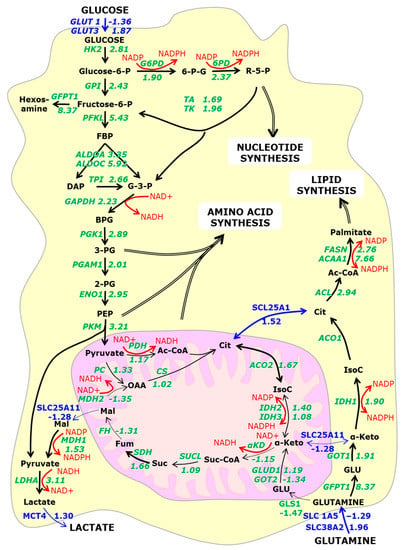The image illustrates the intricate biochemical pathway of glucose metabolism, beginning with the transformation of glucose into glucose-6-phosphate (G6P) and then into fructose-6-phosphate (F6P). The F6P is further converted into fructose-1,6-bisphosphate (FBP) which then splits into dihydroxyacetone phosphate (DAP) and glyceraldehyde-3-phosphate (G3P). The G3P proceeds to become 1,3-bisphosphoglycerate (BPG), followed by several biochemical transformations. Throughout this pathway, the glucose intermediates contribute to various synthesis processes including nucleotide, amino acid, and lipid synthesis, culminating in the production of lactate. Additionally, glutamine is reintegrated into the metabolic cycle. The diagram employs color-coded arrows and text—purples, greens, reds, blues, and blacks—to clearly indicate each step and its associated compounds, emphasizing the complexity of glucose breakdown and its role in metabolic functions, potentially relating to conditions such as diabetes.